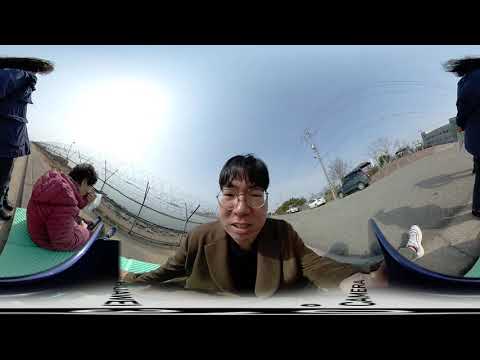This is a panoramic daytime photograph featuring an Asian man with black hair styled in a bowl cut, wearing metal-framed circular glasses, a brown blazer, and a black t-shirt. He is looking directly into the camera with a slightly surprised expression on his face. The panoramic effect gives his face a mildly distorted appearance. 

To his left, there is a person with black hair and glasses, wearing a red puffy ski jacket, partially turned away from the camera. This person is seated on a mint green bench and seems to be either covering their face with their hand or in some form of distress. Behind them, we see a gray street, an industrial chain-link fence with barbed wire, and parked cars including a blue car and two white cars. There's a large lamppost and an electric utility pole in the vicinity, as well as shadows of the people indicating the sunny conditions. The photo has a fisheye-like distortion common with panoramic shots, adding a warped look to the background elements. The sky is mostly blue with the sun visible on the left side.